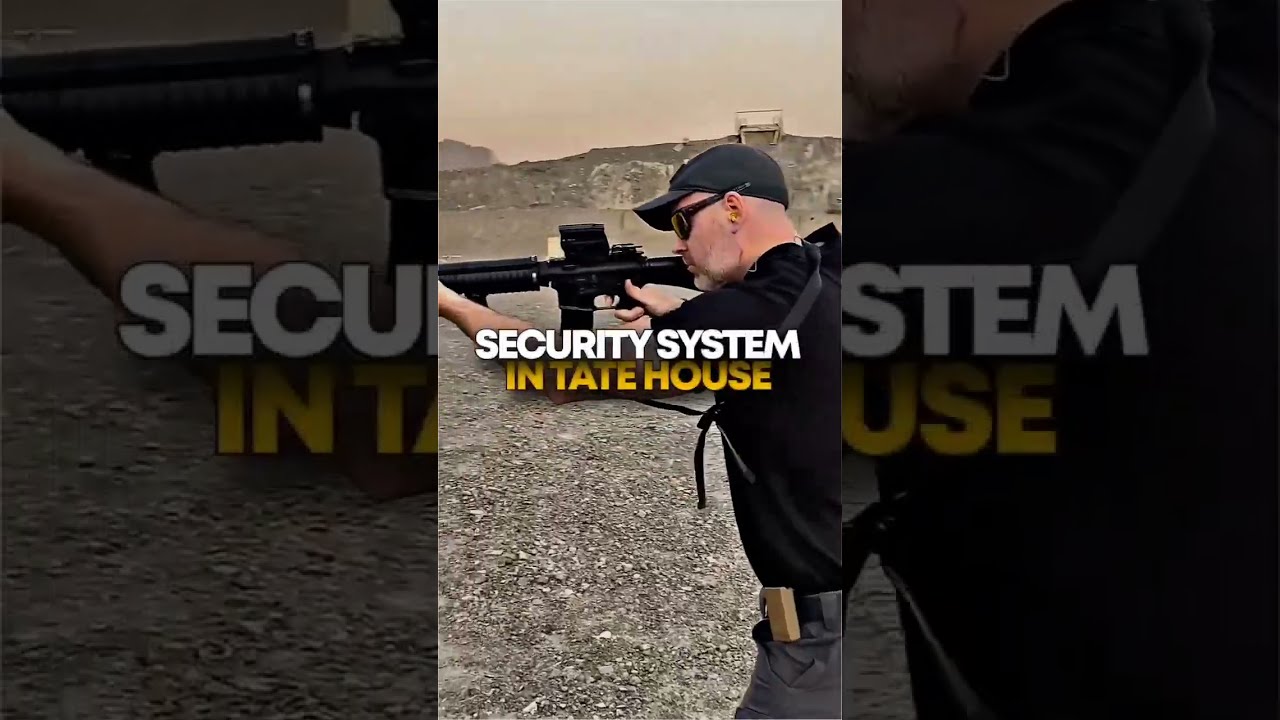The image appears to be a screen capture from a vertical video, possibly from a social media platform like YouTube, Facebook, TikTok, or Instagram. The central image is of a white man at an outdoor shooting range, aiming a black rifle with a scope. He is wearing a black baseball cap and sunglasses, and his tactical yet casual attire includes a black polo shirt and dark cargo pants. The desolate setting features rubble and a gray, gravelly ground with a similarly gray and overcast sky, hinting at a bombed or war-torn area. The text in the image reads "SECURITY SYSTEM" in large white capital letters, with "IN TATE HOUSE" in smaller gold capital letters underneath, both with a shadow effect for emphasis. The composition of the image, with the main vertical photo flanked by echoed, zoomed-in, and faded versions of the same scene on either side, creates a somber and intense atmosphere.